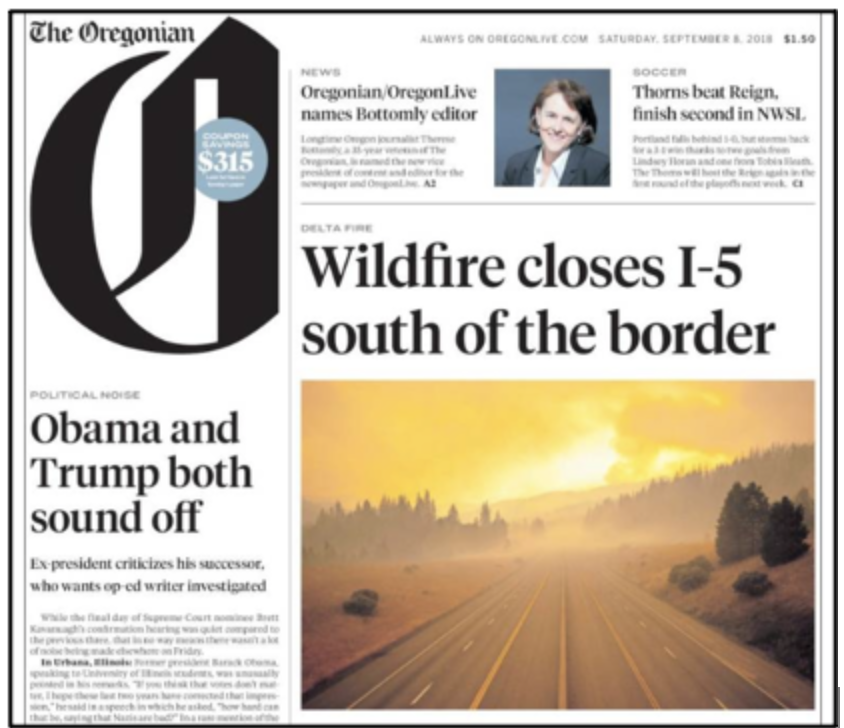An image of the front page of The Oregonian newspaper, dated September 8th, 2018, priced at $1.50, displays the iconic, calligraphy-styled "O" logo prominently at the top. The edition, published on a Saturday, features the website URL "oregonlive.com" under the date. Dominating the center, a major headline reads, "Wildfire closes I-5 south of the border," accompanied by a photograph showing a roadway flanked by forest, with a visible yellowish fire in the distance and smoke billowing into the sky. 

To the left of this main article, a section titled "Political Noise" features commentary on former President Obama and then-President Trump, with several paragraphs elaborating underneath. In the upper right corner, an article announces editorial staff changes with the headline, "Oregonian/Oregon Live Names Bottomley Editor." Below this, a sports announcement declares, "Thorns beat Reign, finish second in NWSL," providing a concise update on recent women's soccer league results.